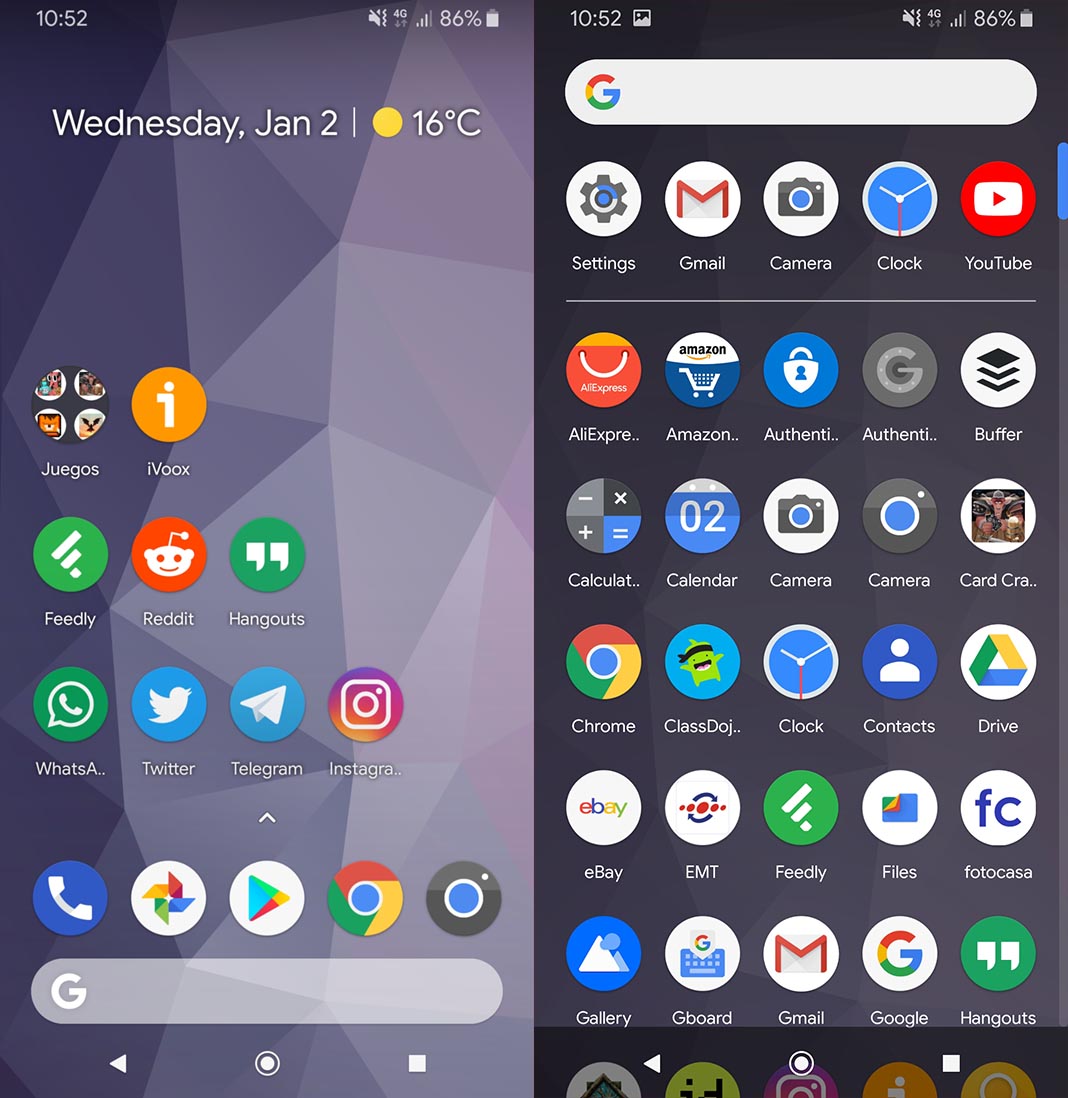Two side-by-side screenshots from an Android device taken at 10:52 AM, showing 86% battery life, 4G connectivity, and three bars of service. 

Left Screenshot:
- Displayed date and time: Wednesday, January 2, 16 degrees Celsius.
- Home screen with multiple apps arranged in four rows.
  - First row: Juegos, iVoox.
  - Second row: Feedly, Reddit, Hangouts.
  - Third row: WhatsApp, Twitter, Telegram, Instagram.
  - Fourth row: Phone, Google Photos, Play Store, Chrome, Camera.
- A Google search bar is located at the bottom of the screen.

Right Screenshot:
- Entire screen filled with app icons arranged in rows, five apps per row.
- Google search bar at the top.
- First row: Settings, Gmail, Camera, Clock, YouTube.
- Additional six rows (at least) filled with various apps, maintaining the five app per row format.